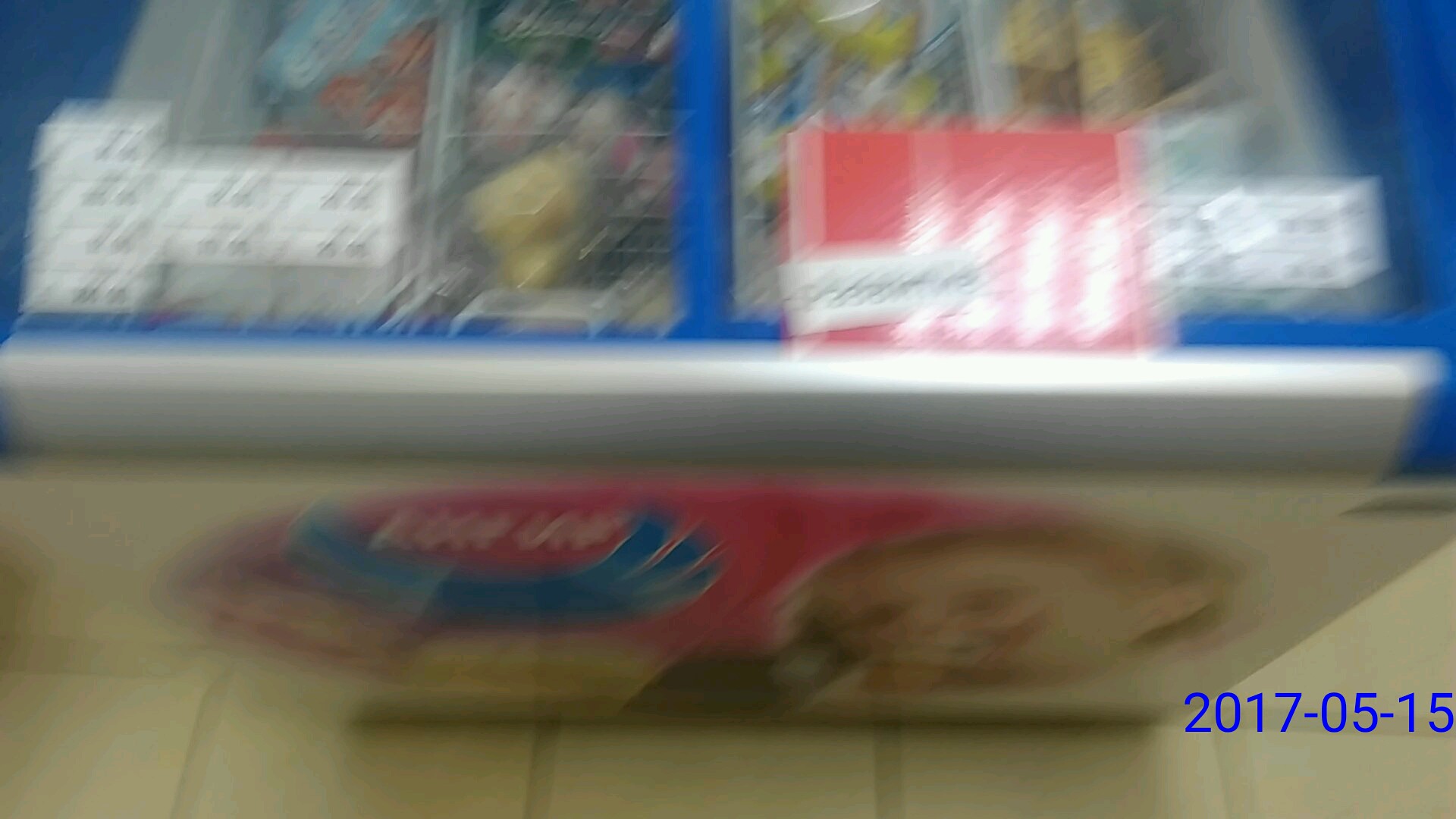The image depicts a blurry ice cream cooler, likely situated in a convenience store or gas station. The cooler has an open-top design with a blue-rimmed lid. The front of the cooler features a pink oval label with a child eating a chocolate ice cream sandwich, next to an indiscernible blue logo. The cooler contains various ice cream products that are too blurry to identify, and there are white stickers and a large red sticker on top. The floor below the cooler is made of beige tile with brown grout. In the bottom right corner, the date "2017-05-15" is displayed in blue lettering.